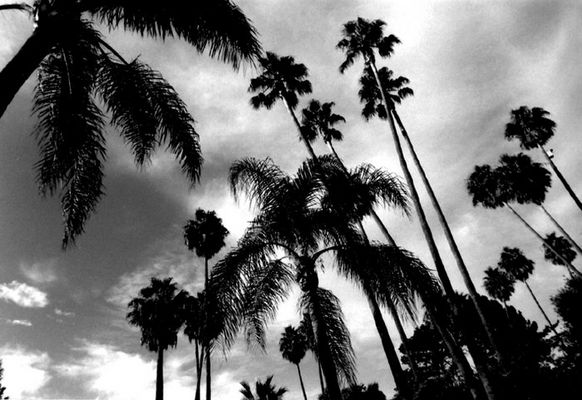This striking black and white photo, taken from a ground-level perspective angled upward, features a variety of tall palm trees set against an overcast sky. The image captures multiple types of palm trees, evident by their distinct shapes and trimming, and highlights coconuts hanging from the central tree. The sky is filled with clouds, appearing gloomy with light peeking through, adding a dramatic effect to the tropical scene. The composition, taken diagonally, includes other types of trees at the edges, enriching the diverse and lush setting.